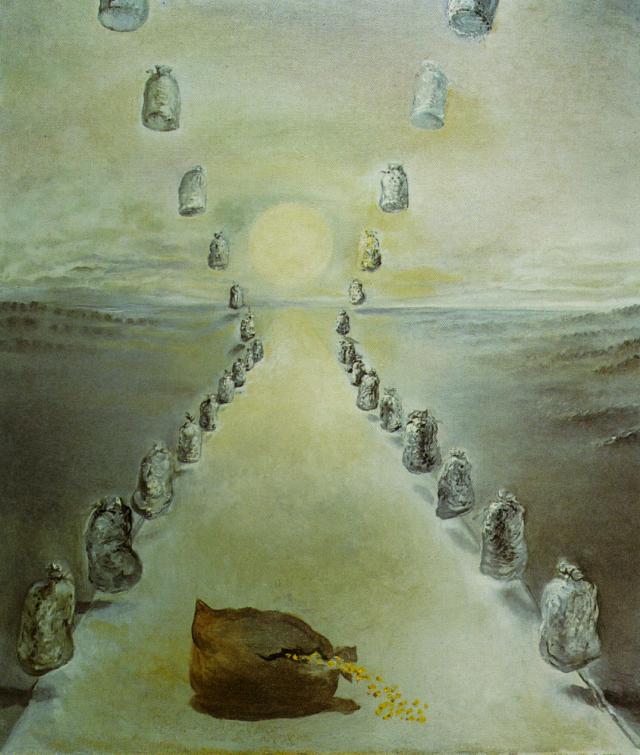In this detailed surrealistic painting, the outdoor setting is dominated by a distant, yellow sun partially obscured by greenish-gray clouds. A bright, white pathway stretches from the foreground to the horizon, directly leading to the sun. Flanking this pathway on either side are a series of gray bags, both on the ground and mirrored in the sky above. The ground surrounding the pathway is described as dark yet slightly foggy, enhancing the dreamlike atmosphere. Notably, in the bottom right corner of the painting, there is a distinctive brown bag different from the others, appearing torn with what looks like golden coins spilling out. This bag contrasts with the gray motif of the other bags. The overall color scheme of the artwork consists of various shades of gray, light gray, white, and stretches of yellow highlights, creating a cohesive and somewhat ethereal landscape.